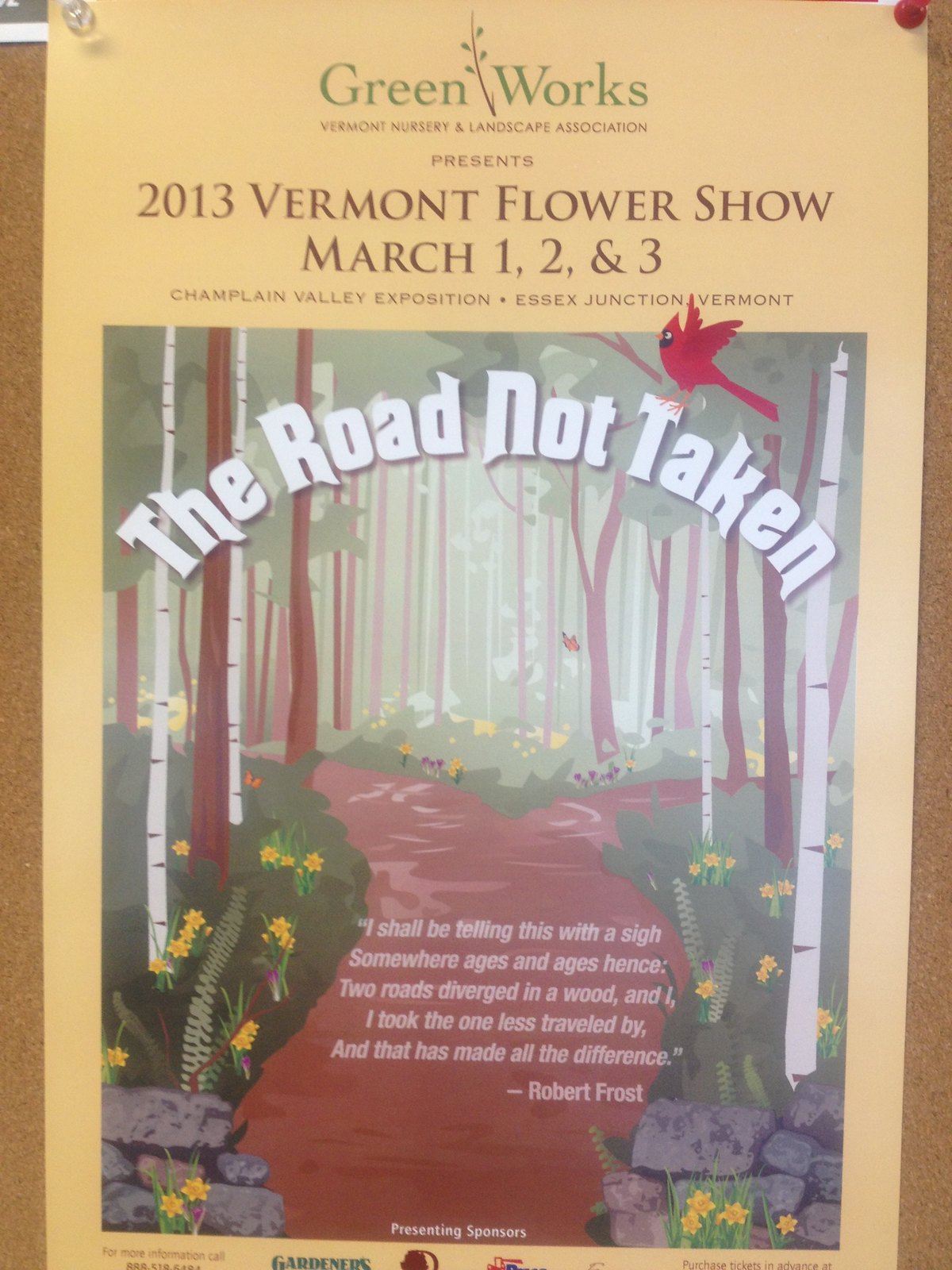This image showcases a poster pinned to a bulletin board using thumbtacks, occupying the majority of the image. The poster advertises the "Green Works, Vermont Nursery and Landscape Association presents 2013 Vermont Flower Show," which will take place on March 1st, 2nd, and 3rd at the Champlain Valley Exposition in Essex Junction, Vermont. The top section of the poster contains this textual information. Below the text, there is a painting depicting a dirt trail winding through a forest and forking to the right midway, accompanied by yellow flowers and stones along the path. Over the painting, the title "The Road Not Taken" is displayed in white letters, with a red cardinal perched on the "T" and rainbow-like arcs above it. Also included is a quote from Robert Frost: "I shall be telling this with a sigh. Somewhere ages and ages hence, two roads diverged in a wood, and I took the one less traveled by, and that has made all the difference." The poster features a palette of colors including brown, tan, green, white, red, yellow, and blue, contributing to its vibrant and inviting appearance. The lower part of the poster mentions "Presenting Sponsors" along with a few sponsor logos, which are not fully visible due to the image cut-off. The detailed design and layout suggest that this is a carefully crafted advertisement promoting both an event and an artistic interpretation of a classic poem.